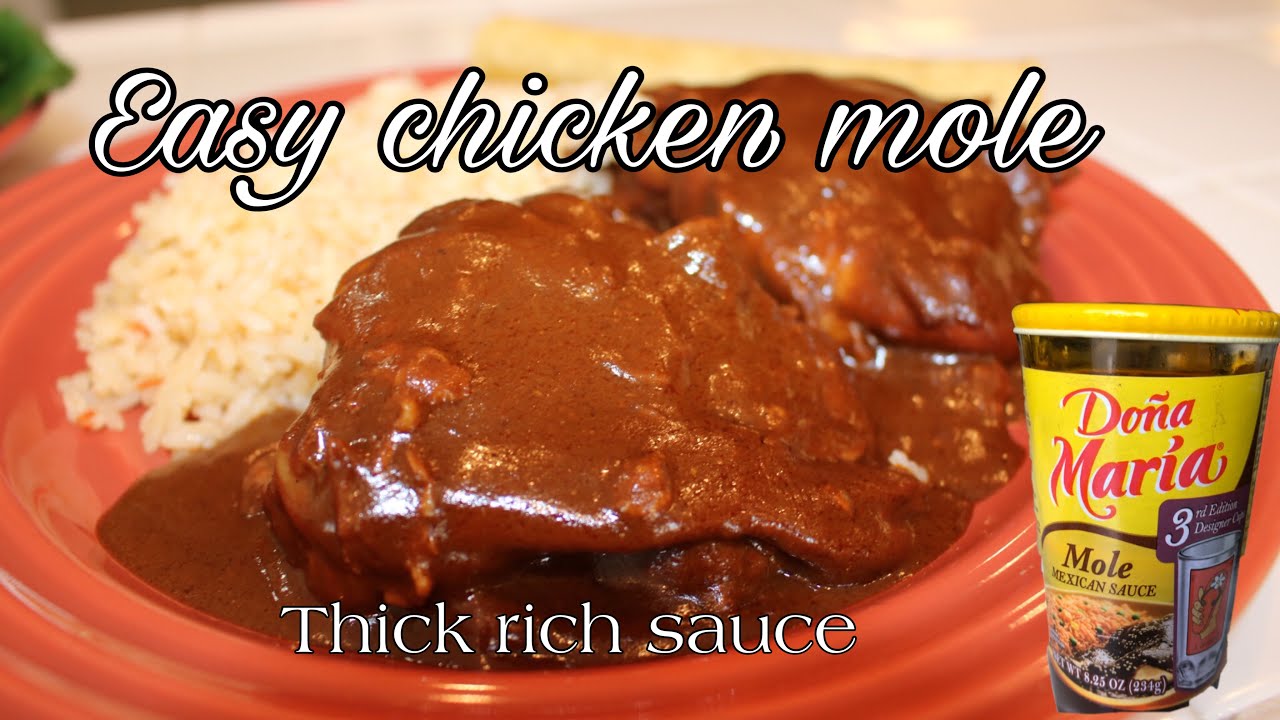This is a detailed promotional image featuring a serving of chicken mole on a plate. The horizontally rectangular photo is digitally enhanced and displayed without a border or background, creating a simple yet engaging presentation. The centerpiece of the image is a pink plate placed on a white surface, holding a portion of chicken covered in thick, rich brown mole sauce, which gives the appearance of steak but is actually chicken. To the side of the chicken is a serving of cooked white rice. 

At the top of the image, superimposed text in white cursive font reads "Easy Chicken Mole," while at the bottom, in regular font, it says "Thick Rich Sauce." In the lower right corner of the image, there is a yellow jar with a flat lid, labeled "Doña Maria" in bold red letters with “Mole Mexican Sauce” in black. The jar also features a picture of food, enhancing the promotional purpose of the image. The overall composition and details suggest that it is a carefully staged photograph designed to showcase the ease and richness of preparing chicken mole using Doña Maria Mole Mexican Sauce.